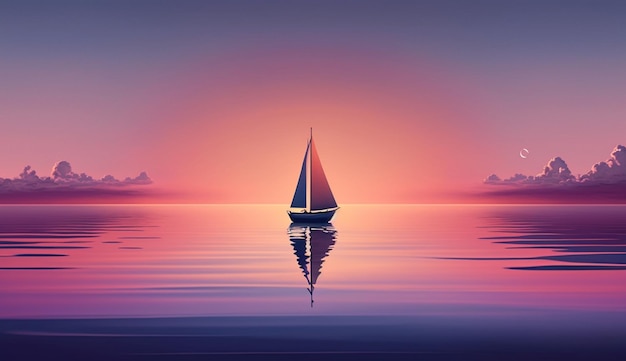A vibrant digital rendering captures a tranquil sunset scene dominated by rich hues of purple, pink, and orange. Central to the image is a small sailboat with two sails—one light orange and the other dark blue—set against the dark blue body of the boat. The boat floats serenely on a rippling body of water, reflecting the sunset’s mesmerizing colors. Above the water's surface, thick gray clouds frame the scene on the left and right sides, with a faint moon or planet peeking out from above the clouds on the right. The sky showcases a rounded, bright pink light, intensifying the sunset's glow, which mirrors off the gently rippled water. The overall composition is a peaceful, almost otherworldly seascape.